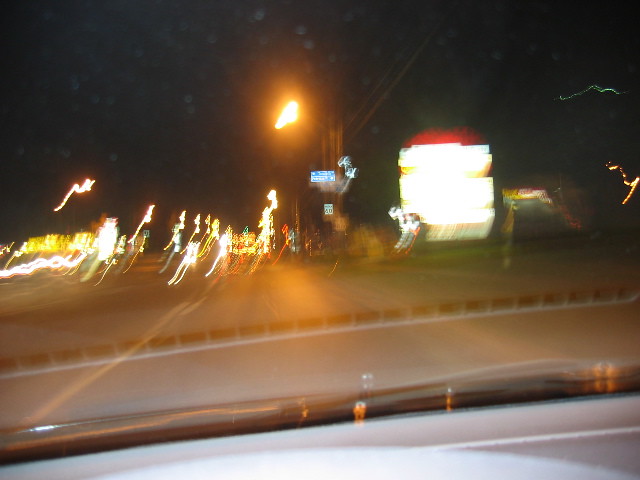A blurry photograph, captured through a dirty windshield, reveals a nocturnal urban scene. Water spots and the reflections of dashboard lights, windshield wipers, and streetlights add to the kaleidoscope of visual elements. The car appears to be in motion, suggested by the streaking lights that illuminate the well-lit thoroughfare. Both sides of the street are adorned with businesses, their neon signs glowing vibrantly yet indistinctly, creating an abstract, almost dreamlike quality. The image encapsulates the dynamic, bustling energy of a city night, albeit through the obscured lens of a moving vehicle.